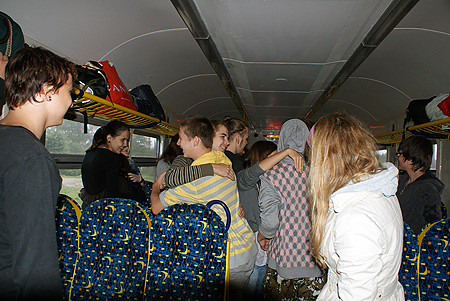The color photograph captures the lively interior of what appears to be an American-style school bus. The bus features a curved, off-white roof and dark navy seats adorned with red, white, and yellow dots, along with some indiscernible yellow symbols. The scene shows a group of high school-aged students standing in the aisle, all smiling and hugging, suggesting a celebratory moment. No one is seated, emphasizing the communal atmosphere. Above the windows, on both sides of the bus, yellow metal racks hold various bags and personal belongings. Notable individuals include a person to the left in a grey sweatshirt with short brown hair, a person in the middle wearing a blue and yellow checkered top with a grey hoodie, and a person to the right in a white coat with blonde hair. The bus exudes a sense of joy and camaraderie, filled with the energy of the students.